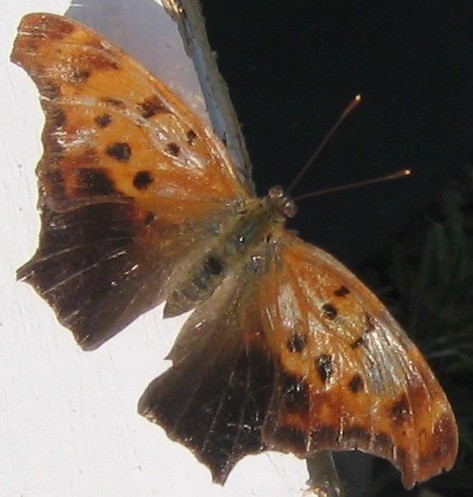This image captures a detailed painting of a moth. The moth, with its body angled down and to the right, exhibits a striking palette of orange wings embellished with black spots. The tips of the wings transition into a stark pitch black, creating a vivid contrast. The moth's body is oval-shaped and gray, with two large antennae projecting diagonally upward from its head. The moth's abdomen tapers down into an almost pointed end, adding to its peculiar appearance. The wings' asymmetry is notable, with each side being similar but not identical.

The background of the painting enhances the moth's striking colors. The left half of the background is predominantly white with a touch of gray paint at the top, intersected by a darker gray diagonal line running from the middle down to the right. The right half transitions into a deep black, suggesting a night-time setting. Dim, almost unrecognizable, images on the right hint at possible plant life, contributing to the enigmatic atmosphere of the artwork. The moth appears to be perched on a surface resembling white wood, further grounding the composition.